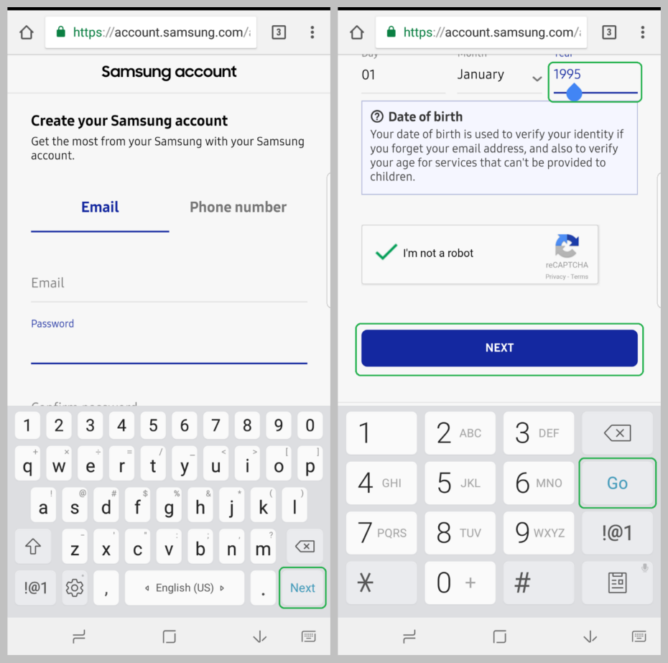**Detailed Caption:**

The image features two side-by-side screenshots of a mobile phone interface for a Samsung Galaxy device, representing the creation process of a Samsung account. 

The first screenshot portrays the initial page for creating a Samsung account. The background is primarily white with black text, while interactive links are highlighted in blue. At the top, the bold header reads "Samsung Account" followed by the subheading "Create your Samsung account" and a brief description, "Get the most from your Samsung with your Samsung account." Below this text, the interface offers two tabs: "Email" and "Phone Number." The "Email" tab is selected and highlighted. Under these tabs, there are two text fields: one designated for entering an email address and the other for a password. Visible at the bottom of this screenshot is the mobile device's keyboard, set to the standard input mode.

The second screenshot on the right captures the subsequent step, where the user inputs their date of birth. The section is labeled "Date of Birth," with the selected date being "January 1995." Below this, there is a small check box for the CAPTCHA verification prompt, labeled "I'm not a robot." Adjacent to this, a prominent "Next" button is displayed, colored blue with white text. Similar to the first screenshot, the lower part of the screen shows the mobile keyboard, here switched to the numeric layout to facilitate easy date entry.